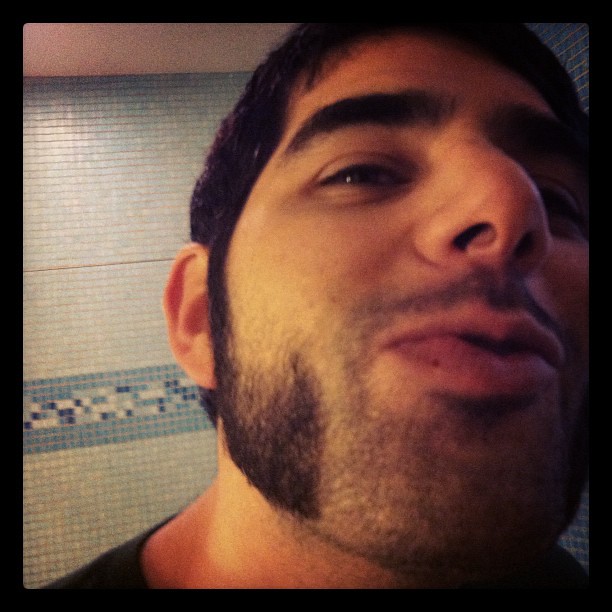This close-up image captures a man with his chin slightly raised, appearing to make a kissy face. He has short, dark black hair and very thick eyebrows that frame his slightly closed eyes. His nose is strong, and his slightly open mouth reveals a Cupid's bow-shaped upper lip. A thin dot is noticeable on his bottom lip. He sports a dark 5 o'clock shadow around his upper lip and chin, which connects to sideburns extending into thick mutton chops that stop just before his chin, leaving a slight stubble on the chin area. The man's dark facial hair contrasts with his complexion, which suggests he might be of Turkish or light-skinned Middle Eastern descent. 

In the background, there is a tiled wall composed of small, light blue square tiles. At the bottom of the image, a darker blue strip runs horizontally, featuring a mix of dark blue, light blue, white, and gray tiles in a decorative pattern. The top edge of a black T-shirt he is wearing is just visible. The overall close proximity of the photo accentuates the details of his facial hair and the intricacies of the tiled wall behind him.